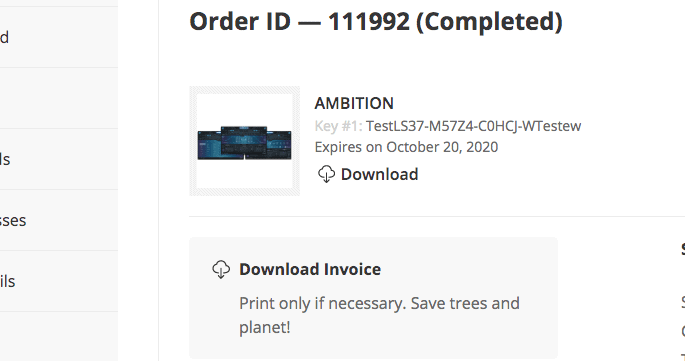This image appears to be a partially cropped screenshot from a website interface, which is divided into two distinct sections. 

In the upper section, the content is organized into six individual boxes. Due to the cropping, some letters and elements are partially visible or entirely cut off. Here's a breakdown of the visible letters:
1. First box: Contains the letter "D."
2. Second box: Completely cut off.
3. Third box: Contains the letters "L-S."
4. Fourth box: Contains the letters "S-E-S."
5. Fifth box: Contains the letters "I-L-S."
6. Sixth box: Completely cut off.

The lower section contains key details about an order. At the top, it displays the text "Order ID - 111992 (Completed)" in bold and larger font. Below this, there is an image depicting three screens—one central and two slightly behind it—framed by a gray box. 

Next to the image is the capitalized word "AMBITION" in black, followed by the phrase "Key Number 1" in gray text. Subsequent information includes an alphanumeric code "test LS-37-M57Z4-C0HCZ-WTESTEW," along with a note that it expires on October 20th, 2020. Below this information, there is a download icon with the label "Download" in black.

Further down, there is another download icon accompanied by the text "Download Invoice" in black. In smaller gray text, it advises to "Print only if necessary, save trees and the planet." Additional details are present but are cut off from the screenshot.

This comprehensive description helps convey the structured nature of the website’s interface and highlights the emphasis on order details and eco-friendly messaging.